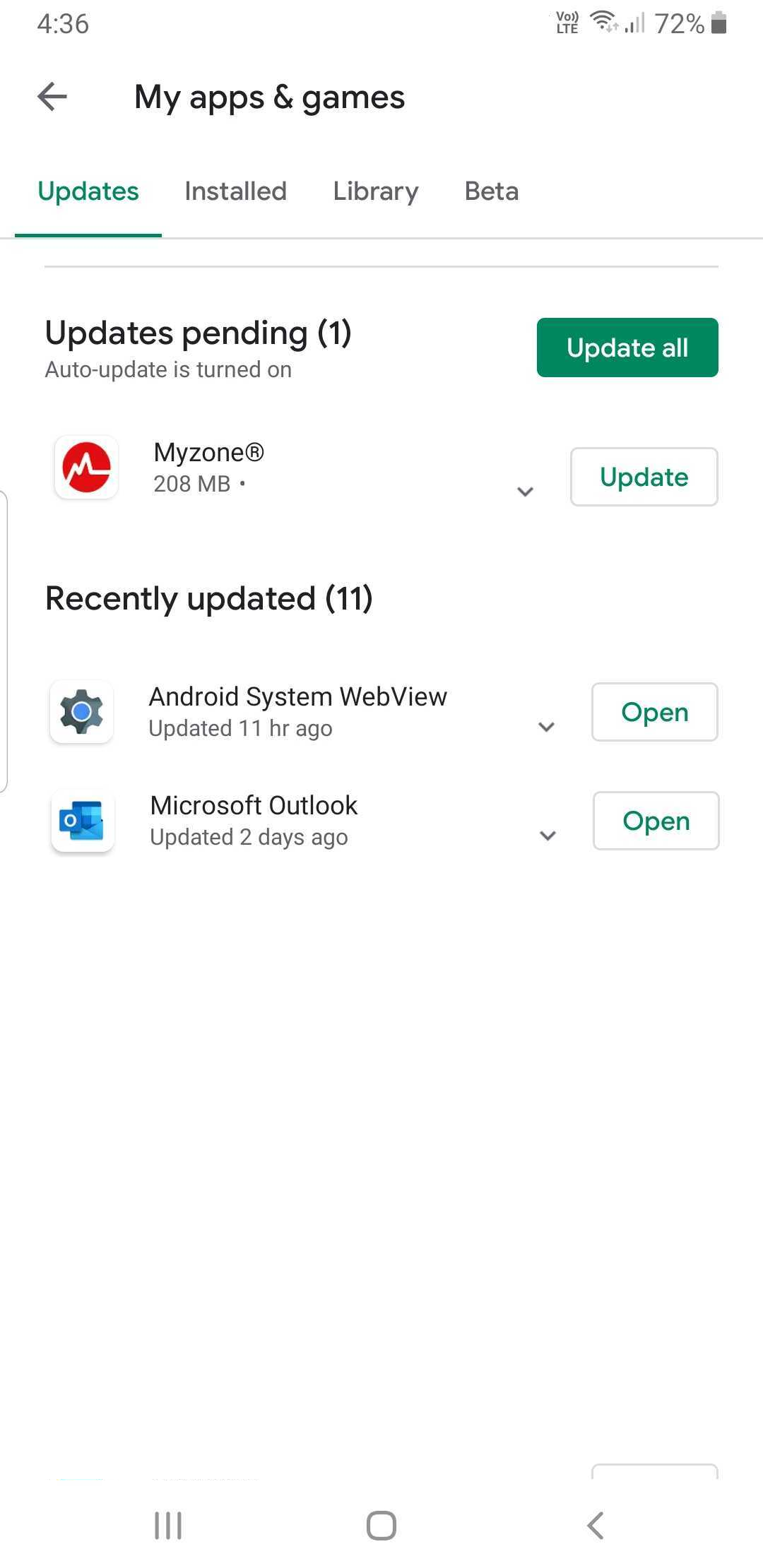The webpage displayed has a predominantly white background with various elements positioned strategically. At the very top, slightly towards the left, the text "My Apps and Games" is written in black. In the upper left corner, the number "436" is also in black lettering. Opposed to this, on the upper right corner, there are several icons indicating battery level, Wi-Fi connectivity, and other status indicators. The battery icon shows a 72% charge in black text.

Just below these status icons, to the left, there's a black arrow pointing to the left with "My Apps and Games" inscribed next to it in black. Below this, the navigation options are displayed, starting with "Updates" in green, followed by "Installed," "Library," and "Beta," each in black text. A green bar highlights the "Updates" section, indicating it is currently selected.

Immediately beneath these navigation options, thin green lines further delineate the sections. The text "Updates Pending" is shown in black with a count of "(1)" in parentheses next to it. Towards the right side of this section, there is a green button labeled "Update All."

In the main content area below this section, two programs are listed: 

1. **Android System WebView** - Positioned to the left, with an option to update on the right.
2. **Microsoft Outlook** - Listed underneath, both have a rectangular green "Open" button to their right, signifying that these programs have been recently updated and can be accessed directly through the button.

Each program entry is accompanied by corresponding symbols and descriptions, allowing users to interact with and manage their applications effectively.